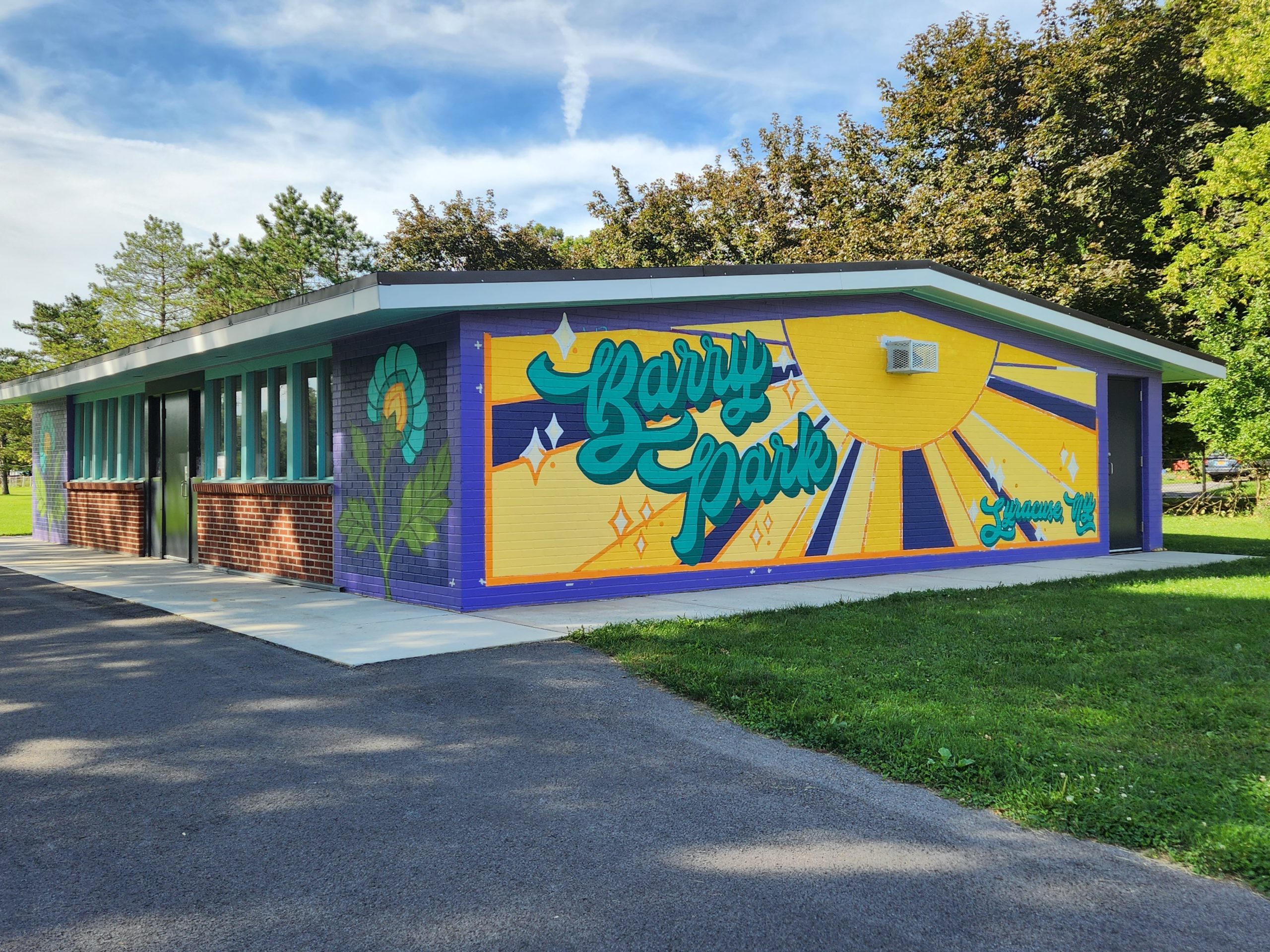The image captures a vibrant, one-story building that's in a park on a sunny day. The front of the building faces the left, featuring a glass door with a black frame, flanked by red brick walls and light blue-framed windows above. The rest of the building is adorned with colorful artwork. On the side of the building that faces the right, there's a large, bright yellow sun drawing and the name "Barrie Park" prominently displayed. The front side also showcases a painted flower with blue petals and green leaves, set against a purple background. The building is surrounded by a concrete walkway and lush grass, leading up to a driveway or parking lot in the foreground. Behind the building, tall trees stretch towards a blue sky dotted with light clouds, adding to the picturesque setting.